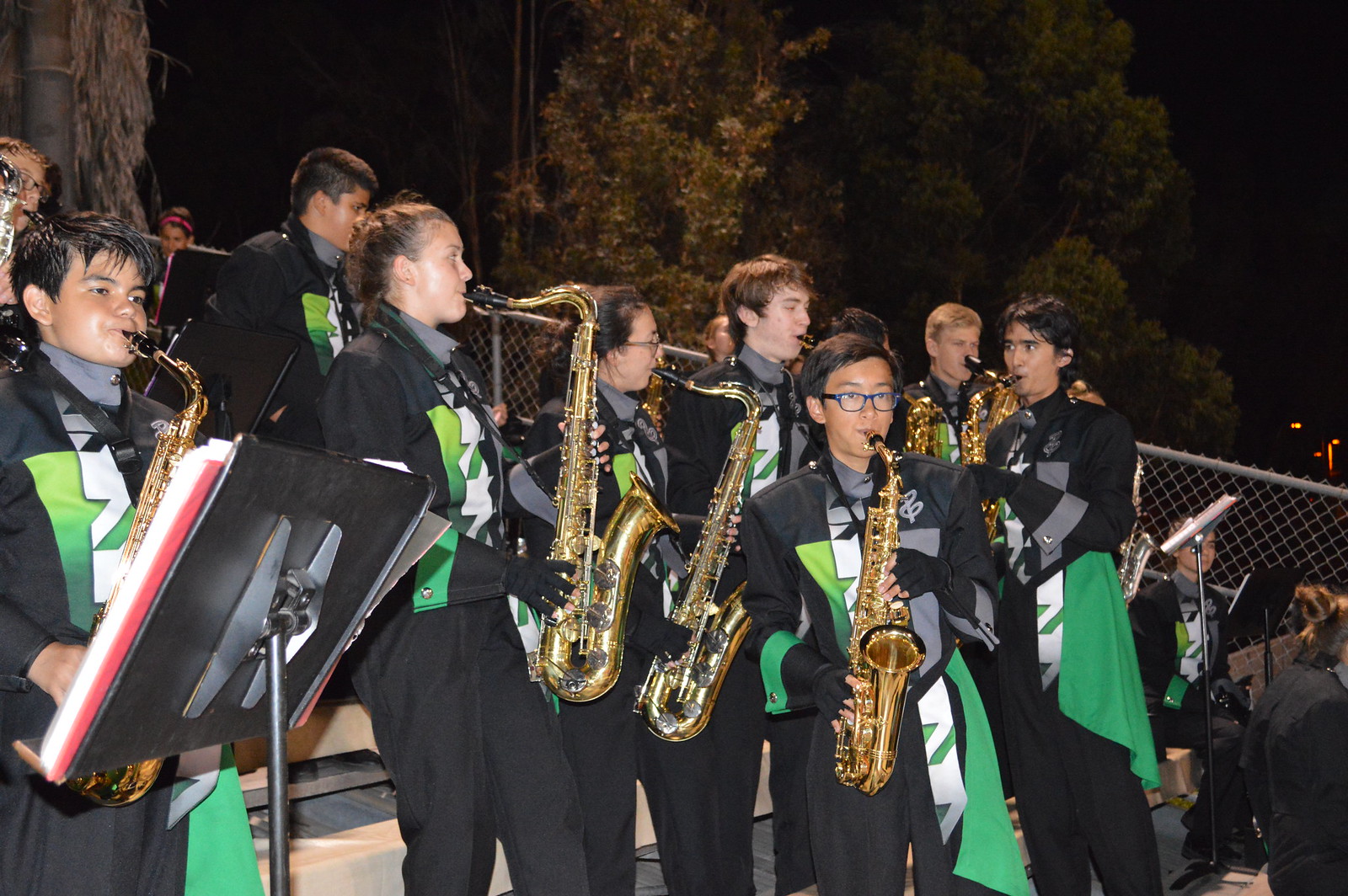This nighttime photograph captures a high school band seated in bleachers, performing under the open sky. The band members are all in uniform, wearing black suits adorned with green accents and subtle white designs along the lapels. Some of them also wear black gauntlet-style gloves with flared cuffs edged in green. The students, with a mix of light skin tones and varying hair colors from dark to blonde, play shiny, gold saxophones. Music stands are scattered among them, holding sheet music steady. The bleachers face to the right, towards an unseen field, with a backdrop of large trees and a metal chain-link fence. The dark night sky sets a dramatic contrast against the band’s uniform colors and the gleaming instruments.